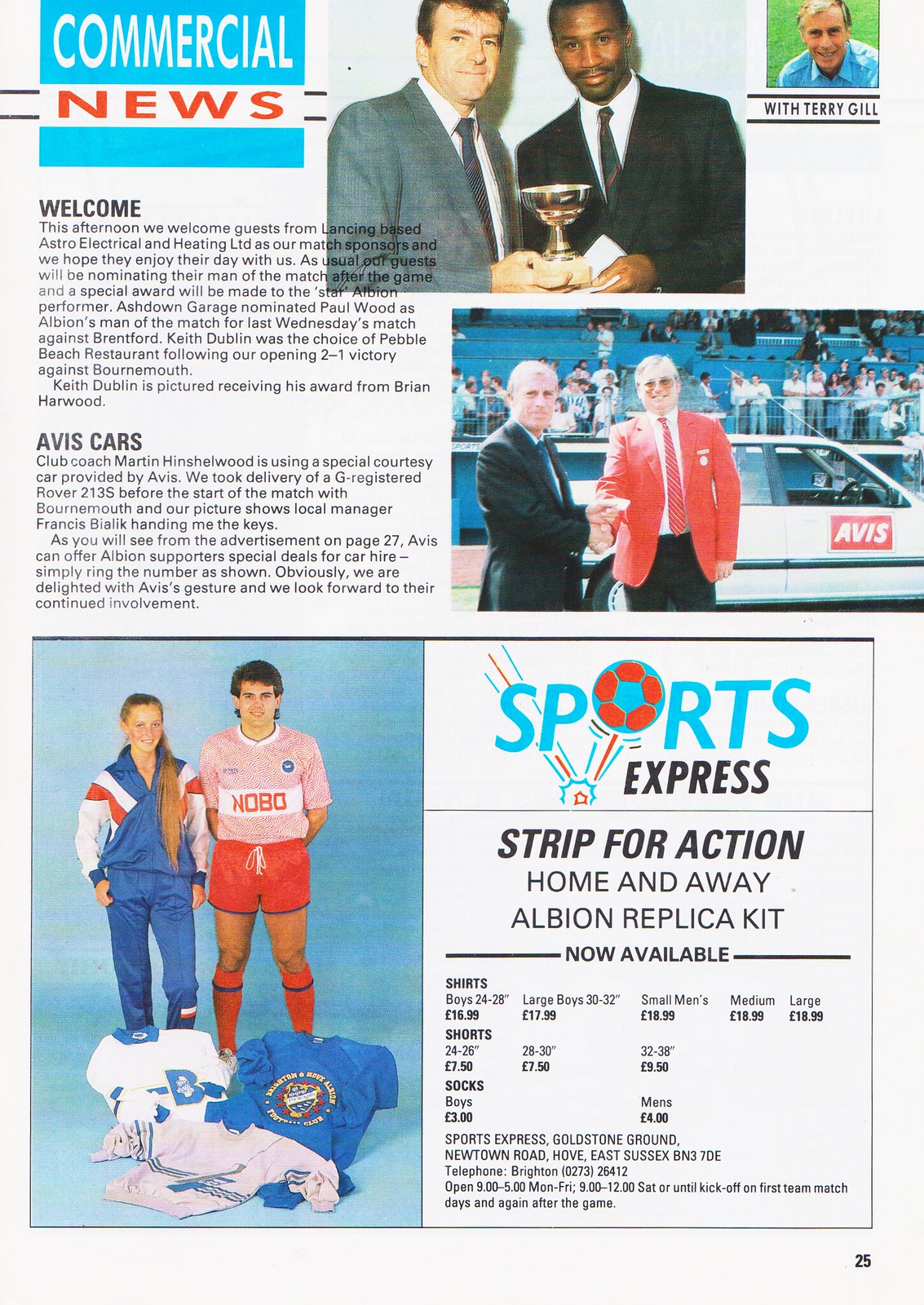**Commercial News, Page 25: A Snapshot of Albion FC's Pride and Partnerships**

The top of the page proudly displays the "Commercial News" title in blue, accentuated with red and white writing. Featured prominently is a photograph capturing a notable moment with two men, one Black and one White, holding a trophy in celebration. To the top right hand corner, Terry Gill is pictured, adding a personal touch to the narrative.

On the left-hand side of the page, the headlines read "Welcome" alongside a paragraph extending a warm invite to guests from Lansing-based Astro Electrical and Heating Limited, who are the match sponsors for the day. As part of their sponsorship duties, these guests will nominate the man of the match. Notably, Ashtown Garage had previously nominated Paul Wood as Albion's man of the match for a game against Brentford, whereas Keith Dublin was the top performer in the 2-1 victory against Bournemouth, receiving his award from Brian Howard.

Further down, Avis Cars gets a mention for their contribution to the club, especially highlighted is the delivery of a courtesy car, a G-Registered Rover 20-213S, presented to coach Martin Hinshelwood by local manager Francis Bialik. The text directs readers to page 27 for special car hire deals for LBN supporters offered by Avis.

In the lower section, the photograph shows the partnership's grassroots reach with visuals of a sponsorship by Sports Express. To the left, a woman in a blue tracksuit stands next to a man donned in a red and white soccer outfit with additional blue, white, and gray jerseys laid out before them, promoting the new Albion Replica Kit. The ad details sizes and prices for boys’, men's jerseys, shorts, and socks, promising gear that fits supporters of all ages.

All of this is encapsulated by guarantees of availability from Goldstown Ground, Newtown Road, Hove, East Sussex, with specified hours and contact information for Brighton supporters, ensuring accessibility to fans near and far.

Overall, this page seamlessly integrates celebration, sponsorship appreciation, and commercial opportunities within the vibrant world of Albion FC.